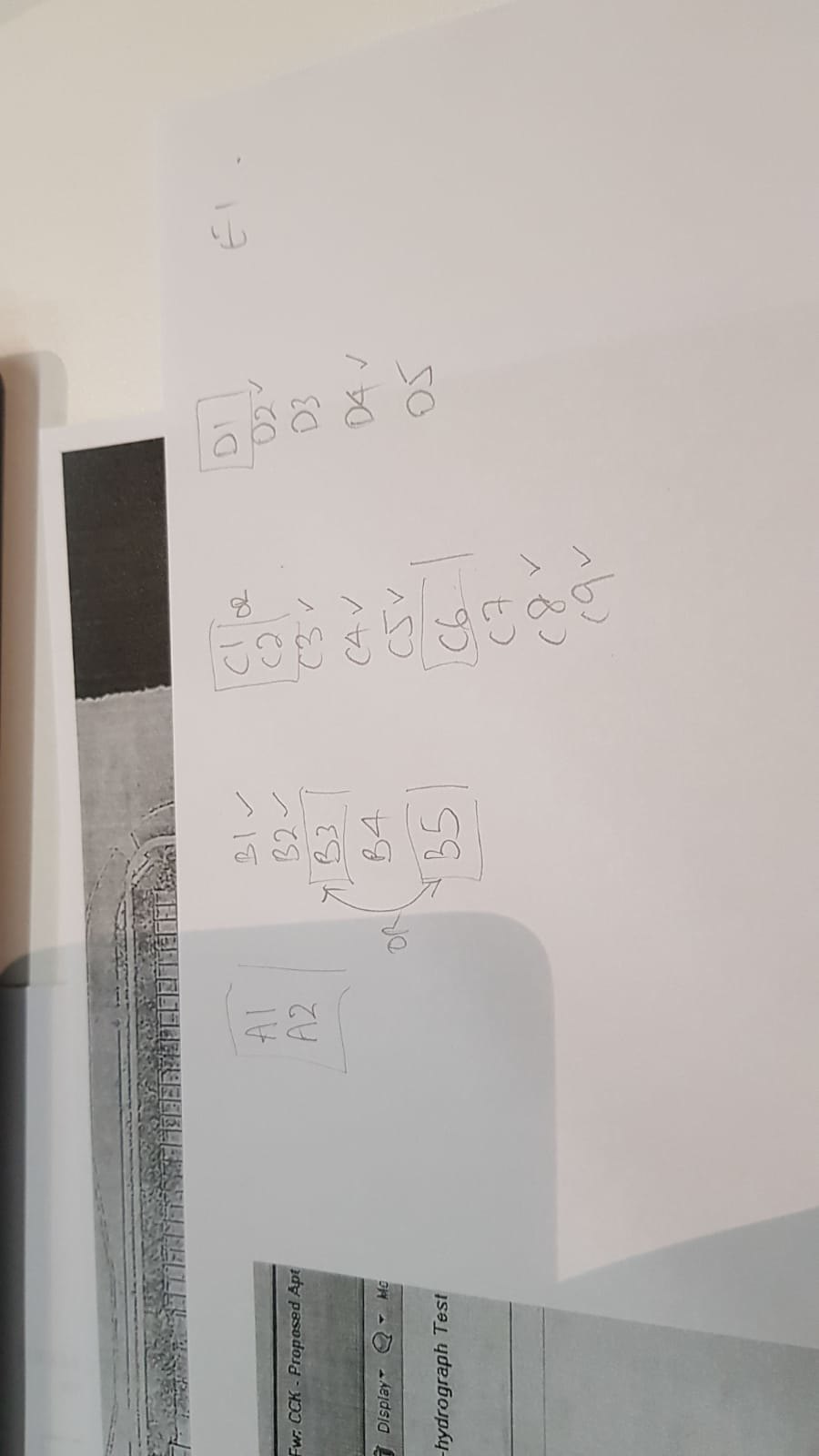The image is oriented vertically, requiring one to tilt their head to the left to view it properly. It depicts a stack of white papers slightly fanned out on what appears to be a desk. The bottom sheet is a photocopy, displaying a grid that is mostly obscured. The second sheet up reveals part of an email, featuring terms like "forward," "CCK," and "proposed APT," which might stand for apartment. The visible section of the email interface includes clickable options like "display," a message bubble icon, several drop-down arrows, and part of the email's subject line, "hydrograph test," printed in black and white. 

The topmost paper shows handwritten notes and various charts in pen. The first column lists items A1 and A2, separated by the word "or." Another column lists items B1 through B5, where B3 and B5 have arrows pointing to them. B4 is unmarked, while B1 and B2 have checkmarks. A third column lists C1 through C9, with C1 and C2 enclosed in squares. C6 is boxed in a rectangle, and C7 has no markings. C1, C2, C3, C4, C5, C8, and C9 feature checkmarks, while C7 remains untouched and is written in a European style. A final column lists D1 through D5, with D1 boxed and D2 and D4 checkmarked. An unfinished column begins with E1. The diagram appears to be a comparative chart, likely used to evaluate different aspects of the hydrograph test.